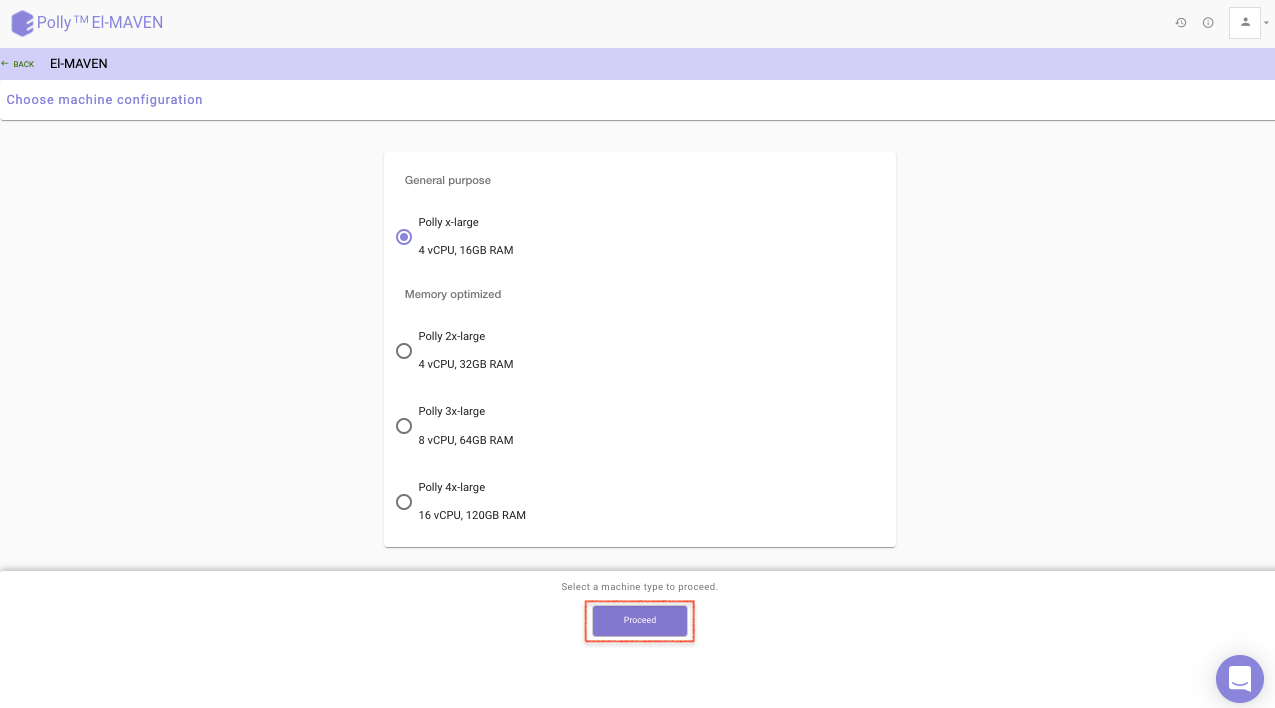Screenshot Description:

This screenshot captures a settings pop-up on a computer screen with multiple elements. 

- **Top Bar:**
  - **Upper Left Corner:** Displays the text "Poly L Maven" prominently.
  - **Upper Right Corner:** Features a back button (or possibly a redo button), an info button, and a profile box with a drop-down arrow.

- **Second Row:**
  - A prominent purple bar stretches horizontally across the page.
  - On the far left side of this bar, there is a green arrow pointing to the left labeled "Back" in green text, indicating the back button.
  - To the right of the green arrow, the text "L Maven" appears in black letters. The rest of the row is devoid of any other elements.

- **Content Area:**
  - The next row begins with the text "Choose Machine Configuration" displayed in purple letters on the left side.
  - Below this, a list of machine configurations is provided:
    - General Purpose
    - Poly Extra Large
    - Memory Optimized
    - Poly 2x Large
    - Poly 3x Large
    - Poly 4x Large

- **Bottom Section:**
  - At the very bottom of the pop-up, there is a large purple "Proceed" button.

This detailed layout aids users in configuring machine settings efficiently, guiding them through various options and ensuring easy navigation back to previous screens.